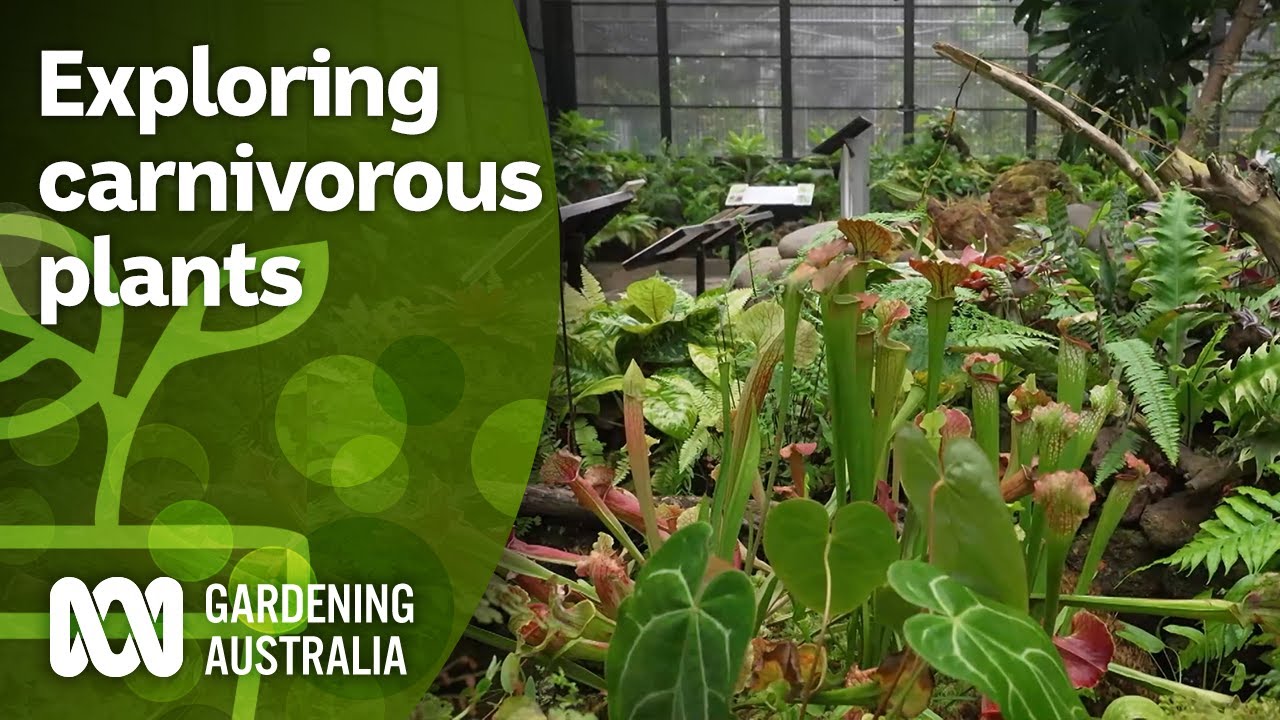The image is a detailed poster, predominantly divided into two sections, promoting the exploration of carnivorous plants with the headline "Exploring Carnivorous Plants" and "Gardening Australia" at the bottom left accompanied by an interlocking white logo resembling an "M" and "W" or a spring. The left side of the poster features a green background with plant illustrations and descriptive text. The right side showcases a vivid photograph of an indoor greenhouse filled with a variety of exotic plants, including prominent deep green leaves, tube-like insect-eating plants, ferns, and placards describing each type. The background displays white steel structures that suggest walkways or stands for additional information on the plants, creating an inviting visual for plant enthusiasts.